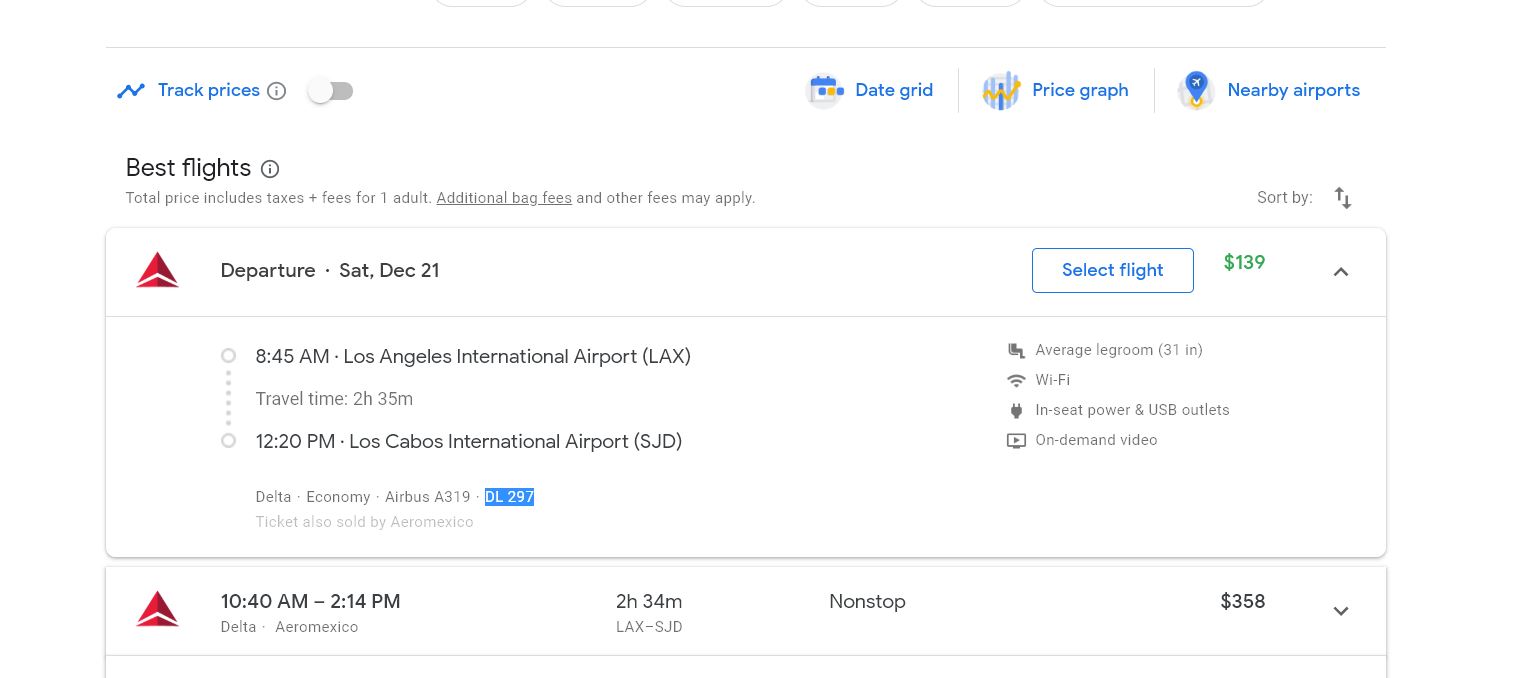The image showcases a primarily white webpage with various sections and black text. Some elements are highlighted with color for emphasis, including blue text and colorful icons. 

In the upper left corner, blue text reads "Track prices" accompanied by a toggle button, which is currently grayed out. To the right, there's a navigation bar with blue text options labeled "Date grid," "Price graph," and "Nearby airports." 

Below this navigation bar, a section titled "Best flights" provides detailed information about flight options. It includes a note that the total price incorporates taxes and fees for one adult, with potential additional baggage and other fees. Adjacent to this section is a "Sort by" button featuring an up and down arrow.

Two flight options are prominently displayed. The first flight option lists:
- Departure: Saturday, December 21st
- Time: 8:45 AM
- From: Los Angeles International Airport (LAX)
- Travel Time: 2 hours and 35 minutes
- To: Los Cabos International Airport (SJD)
- Price: $139
A "Select flight" button with blue text on a white background is available for this flight.

The second flight option provides further information:
- Departure Time: 10:40 AM
- Arrival Time: 2:14 PM
- Trip Duration: 2 hours and 34 minutes, nonstop
- Price: $358